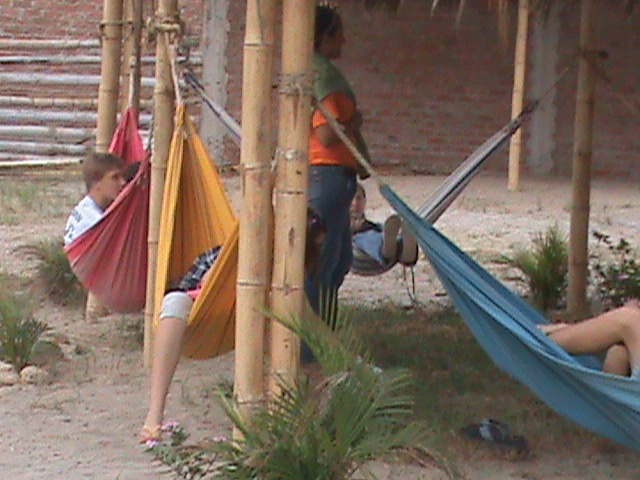The photograph captures a lively scene in a tropical setting with tan, sandy ground dotted sporadically with small palm plants. In the center, a square formation of large-diameter, light-brown bamboo posts, firmly anchored in the ground, supports a series of four colorful cloth hammocks. From left to right, there's a red hammock, a yellow hammock beneath it, and a blue hammock to the right. Each hammock cradles a small child, aged approximately 10 to 12 years old. The child in the red hammock is visible with brown hair and a white t-shirt. The yellow hammock holds another child whose leg is peeking out, while the occupant of the blue hammock is also partly visible, with only their legs showing. In the background, a red brick building provides a rustic backdrop. To the left, behind the main focus of the image, stands a large wooden gate constructed from tree trunks. A woman, dressed in an orange t-shirt and blue jeans, stands casually near the hammocks, adding a touch of everyday life to this picturesque scene.